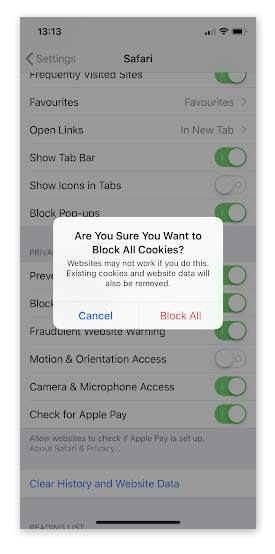The image is a detailed screenshot taken from a smartphone, displaying a specific time of 13:13 in military time at the upper left-hand corner. The screen shows the settings page for the Safari web browser app. Prominently featured in the foreground is a pop-up message that reads: "Are you sure you want to block all cookies? Websites may not work if you do this. Existing cookies and website data will also be removed." This pop-up provides two options— a "Cancel" button, highlighted in blue text, and a "Block All" button, emphasized in red text.

In the background, the Safari settings page is visible, including various configurable options such as "Frequently Visited Sites," "Favorites," "Open Links," "Show Tab Bar," "Show Icons in Tabs," and "Block Pop-ups." Each of these settings has a toggle switch on the right side, which can be either green (indicating the feature is enabled) or white (indicating the feature is disabled). The screenshot captures a comprehensive overview of this settings interface in a smartphone display.